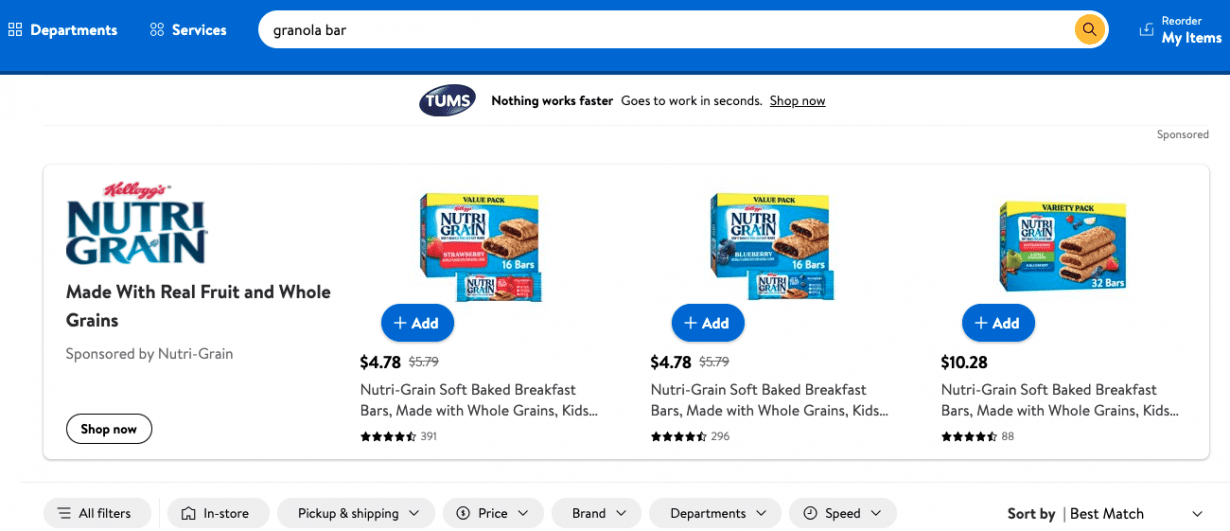Screenshot of an online shopping page for Kellogg's Nutri-Grain bars:

The screenshot captures an online shopping page showcasing three options for Kellogg's Nutri-Grain bars, presented with vibrant color images of the product and its retail packaging. Each product box prominently features a yellow bar at the top indicating it is a "value pack." The front of each box displays illustrations of the bars along with the specific flavor.

1. **Strawberry Filling:** The first option features a strawberry filling.
2. **Blueberry Filling:** The second option displays a blueberry filling.
3. **Mixed Flavor Pack:** The third option is a mixed flavor pack, containing a variety of flavors.

Below the images of each product, there are small blue buttons with white text labeled "Add," which users can click to add the item to their online shopping cart. The prices for each retail package are listed below these buttons. The first two options show a sales price with the original price crossed out, indicating savings. The third option, the mixed pack, contains twice as many bars as the other two and is priced higher.

Directly below each product, there are truncated text descriptions detailing the contents of the boxes. Each product also includes a row with star ratings and the number of reviews left by customers.

At the very bottom of the screenshot, there are additional dropdown menu options for further customization: "All filters," "In-store," "Pickup & shipping," "Price," "Brand," "Departments," "Speed," and "Sort by" with a dropdown displaying "Best match."

The top of the page features a blue bar with clickable sections labeled "Departments" and "Services," followed by a large white search bar with a yellow circular search icon. At the end of this blue bar, there is small text labeled "Reorder," and below that, in white text, it reads "My items."